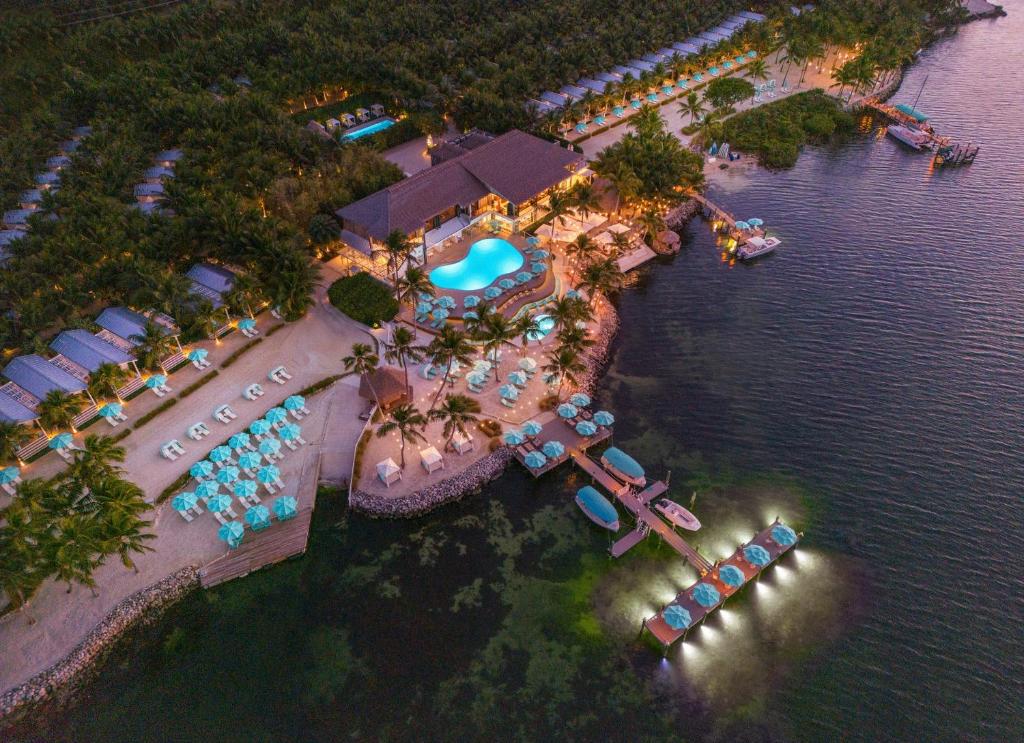This serene outdoor image captures a luxurious resort setting by the water. Dominating the scene is a uniquely shaped pool, reminiscent of a peanut, with a bright turquoise blue color and subtle ripples on its right side. Surrounding the pool are numerous chairs and light blue umbrellas, set up against a backdrop of lush palm trees and other foliage, enhancing the tropical ambiance. Adjacent to the pool stands a building with a brown rooftop, hinting at a pool house or part of the resort complex. The presence of lights suggests an inviting, illuminated atmosphere, likely part of a hotel or resort complex that's perfect for relaxation and leisure.